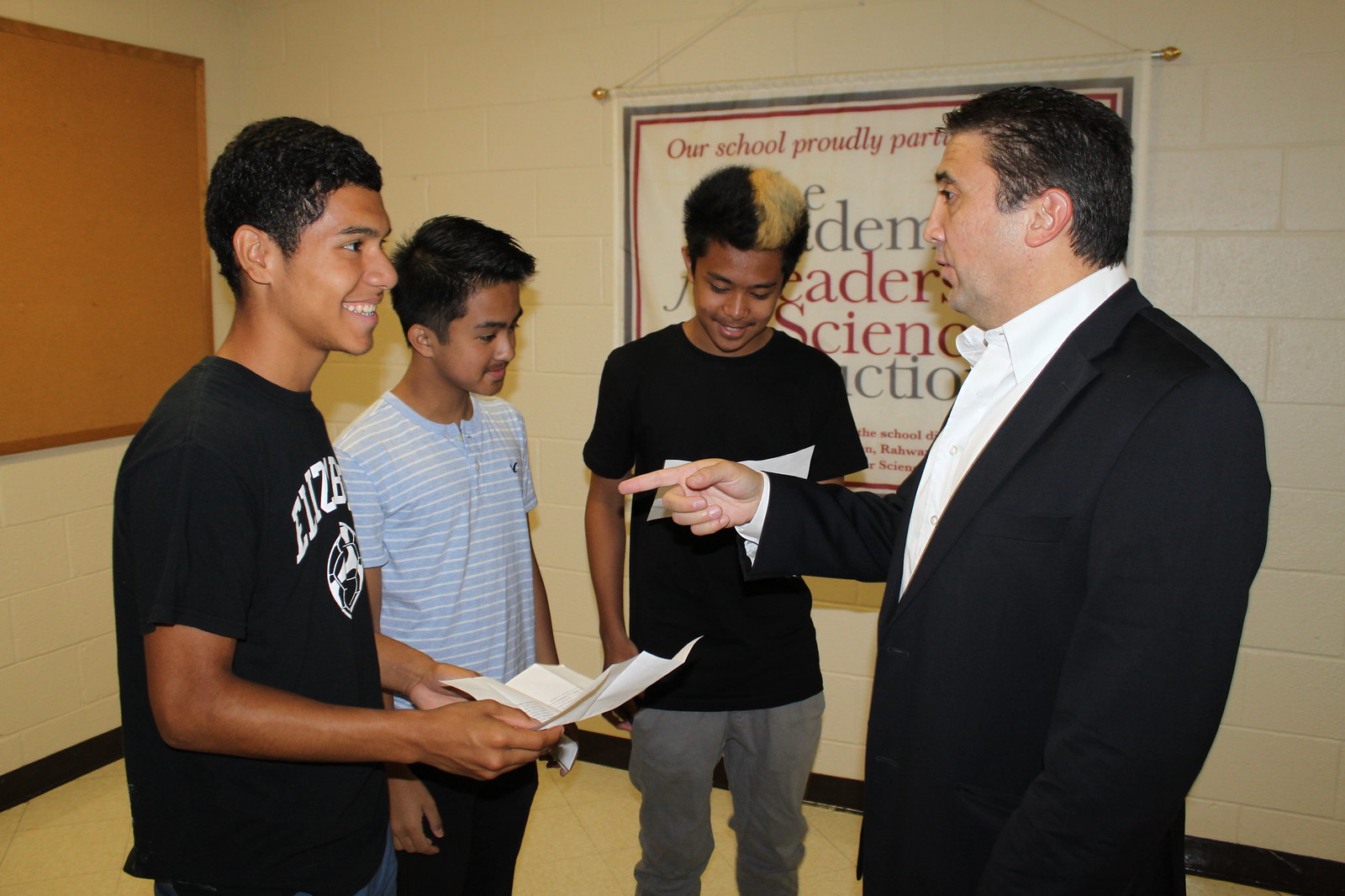In this photograph taken in a school hallway, an adult man with short black hair, likely in his late 40s, is engaging in a conversation with three high school students. The man is dressed in a black sport coat over a long-sleeved white shirt, without a tie, and is pointing towards one of the boys. The three students appear to be Latino and have light brown skin. The boy being pointed at is wearing a black t-shirt with a football image on it, smiling, and holding an unfolded piece of paper. To his right, stands a boy in a baby blue shirt with white stripes, looking at the paper the first boy is holding. The third boy, on the far right, has a distinctive half-black, half-white dyed afro, is dressed in a black t-shirt and gray pants, and is also holding a white paper. In the background, there is a sign on the wall that reads, "Our School Proudly Partakes..." followed by some obscured text. The scene conveys an informal yet engaging interaction likely centered around the papers the students are holding.